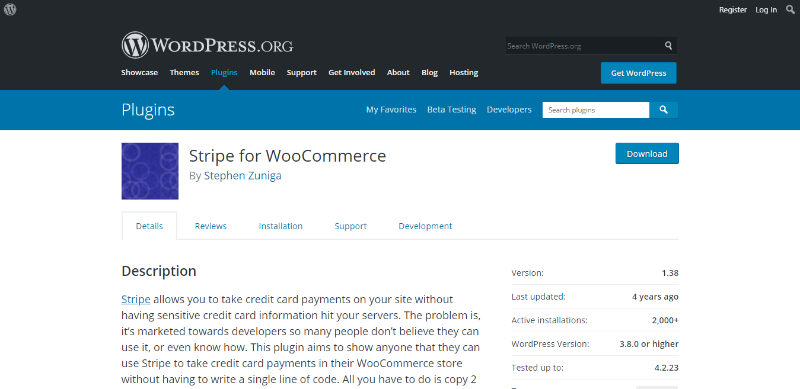This image is a screenshot of the WordPress.org website featuring its plugins section. The top of the site is set against a black background with the WordPress logo and "WordPress.org" written in white text. Below this, a navigation menu lists options such as Showcase, Themes, Plugins, Mobile, Support, Get Involved, About, Blog, and Hosting, with "Plugins" currently highlighted.

Directly beneath the navigation menu, a blue horizontal rectangle stretches across the page displaying the word "Plugins" in white text. To its right, there are additional options: My Favorites, Beta Testing, and Developers, along with a white search box.

Further down, the page features a purple square with a faded round design. To the right is a detailed plugin entry. In gray text, the entry is titled "Stripe for WooCommerce by Steven Zuniga." A blue "Download" button is located immediately to the right.

Below the plugin title area are several tabs labeled Details, Reviews, Installation, Support, and Development, all in blue text. The Details tab currently shows a description stating: "Stripe allows you to take credit card payments on your site without having sensitive credit card information hit your servers. The problem is it's marketed towards developers, so many people don't believe they can use it or even know how. This plugin aims to show anyone that they can use Stripe to take credit card payments in their WooCommerce store without having to write a single line of code. All you have to do is copy to."

To the right of the description is the plugin’s meta-information, including version 1.38, last updated four years ago. The data reveals 2,000 active installations and supports WordPress versions 3.8.0 or higher, tested up to 4.2.23.